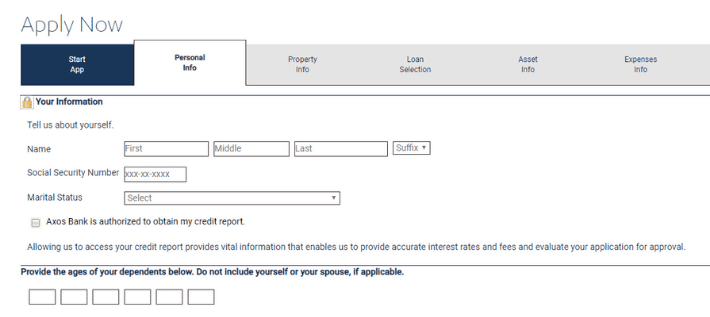A detailed webpage displays a form for filling out personal information, with various sections and tabs for a comprehensive application process.

At the top of the form, there is a tab labeled "Apply Now" indicating the initial stage has already been completed. The current section, "Personal Info," is highlighted with a white tab, positioned to the left of several other sections: "Property Info," "Loan Selection," "Asset Info," and "Expenses Info." These tabs are distinguished by a blue color.

The page is titled "Your Information" in a bold, blue font at the bottom tri-section, focusing on personal details. To the left of the title, an icon of a lock is visible, symbolizing that the information is secure.

Below the heading, a section prompts users to "Tell us about yourself." This includes fields for entering one's first, middle, and last names, along with a suffix option (Mr., Mrs., etc.). Following this, there are input fields for Social Security numbers and marital status, which can be selected from a dropdown box.

Additionally, there is a checkbox option labeled "Axos Bank is authorized to obtain my credit report." This option is currently unchecked. Below this, an explanatory note in bold, blue text states, "Allow us to access your credit report; it provides vital information enabling us to provide accurate interest rates, fees, and evaluate your application for approval."

Further down the page, a horizontal line spans the width of the form, marking a new section. The bold blue text under this line instructs applicants to "Provide the age of your dependents below. Do not include yourself or your spouse if applicable."

Overall, the form utilizes a combination of blue and bolded text to emphasize important details and guide users through the application process smoothly.